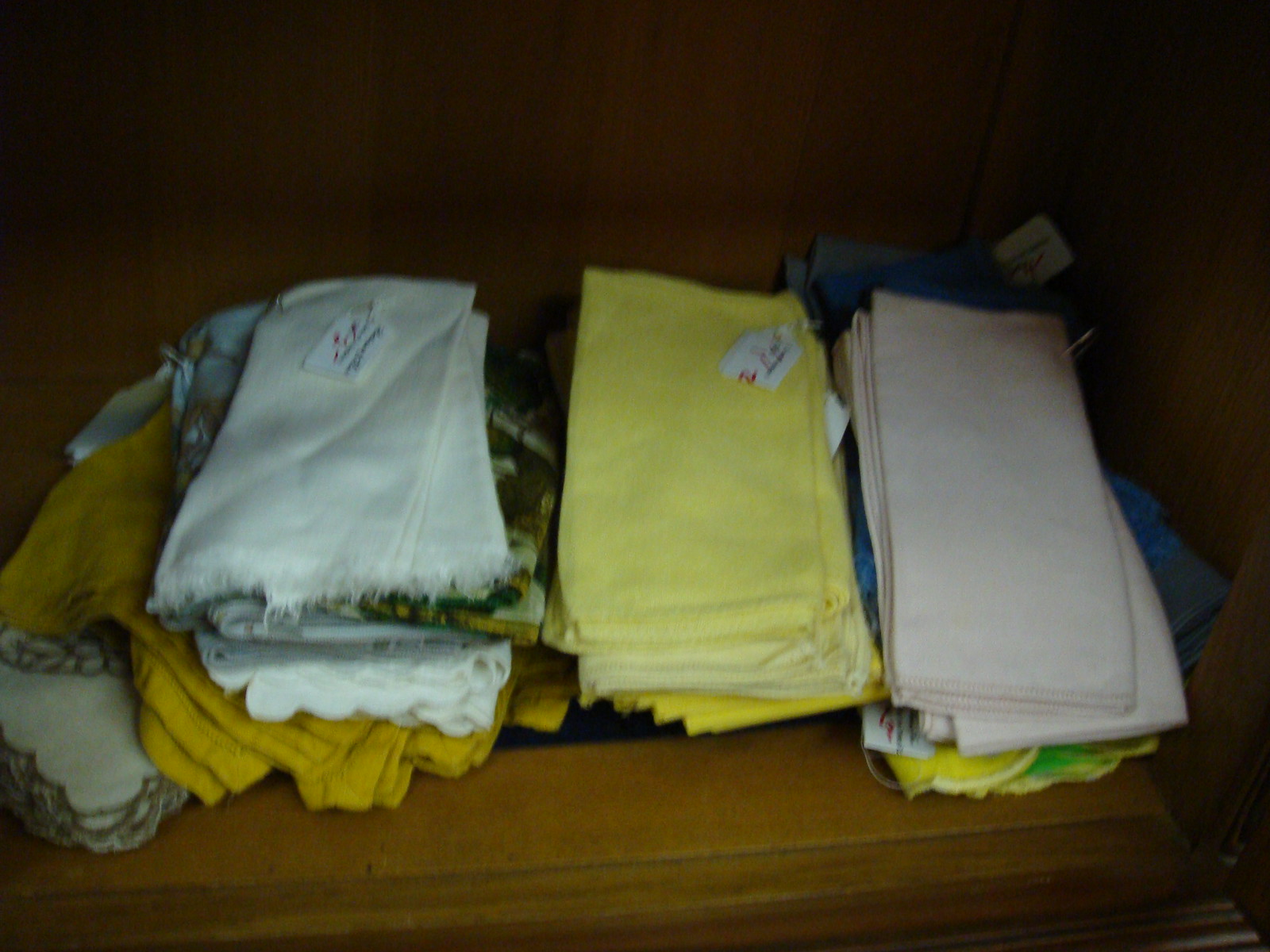In the image, we see a countertop made of light-colored wood, possibly maple, adorned with neatly folded cloths. These cloths appear to be hand towels, arranged into three distinct piles. Each pile showcases a variety of colors, including plain whites, various shades of yellow—from light to mustard—and pale pinks, with hints of blues and greens peeking out from the bottom layers. The cloths are uniformly folded into rectangles. Visible on the top of each stack, a few have white price tags, suggesting they might be for sale, perhaps at a garage sale. The overall setting gives off a vintage vibe, reminiscent of older, more traditional wooden furniture.